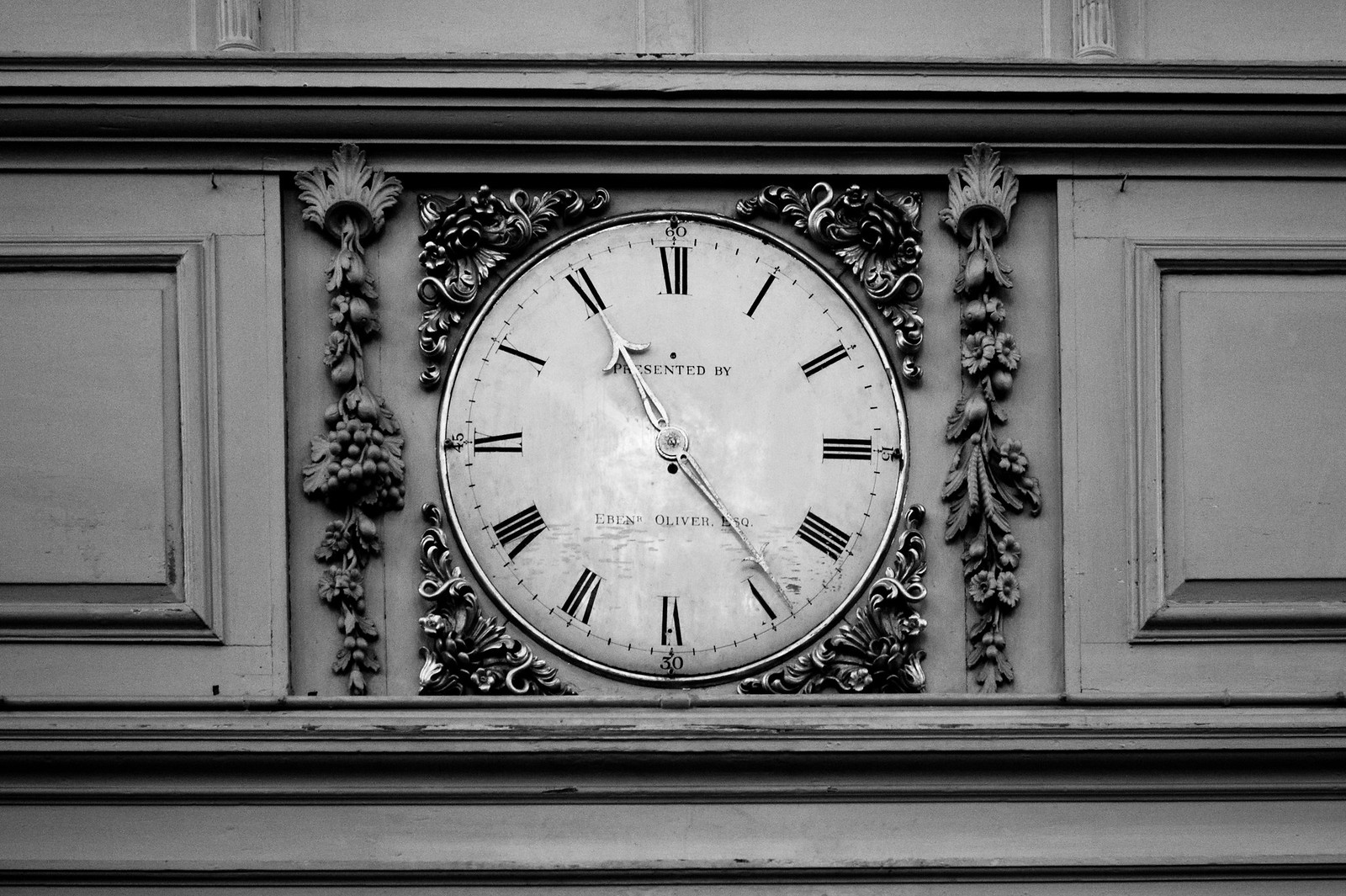This monochrome photograph captures a large, intricately designed clock mounted on what appears to be the side of a building or possibly a door. The entire image is rendered in shades of black and gray, accentuating the vintage aura of the clock. The clock face is adorned with traditional black Roman numerals and bears an inscription at its center reading "Presented by Eben Oliver," with an additional detail partially obscured by the minute hand. The clock shows the time as 11:24, with the hour hand pointing to 11 and the minute hand just shy of 5. Surrounding the clock is an ornate floral design, adding an element of elegance. The clock is set against a wooden background, composed of various square patterns and grooves, suggesting a meticulously crafted door or paneling behind it. This artistic interplay of textures and designs enhances the historical and decorative charm of the scene.